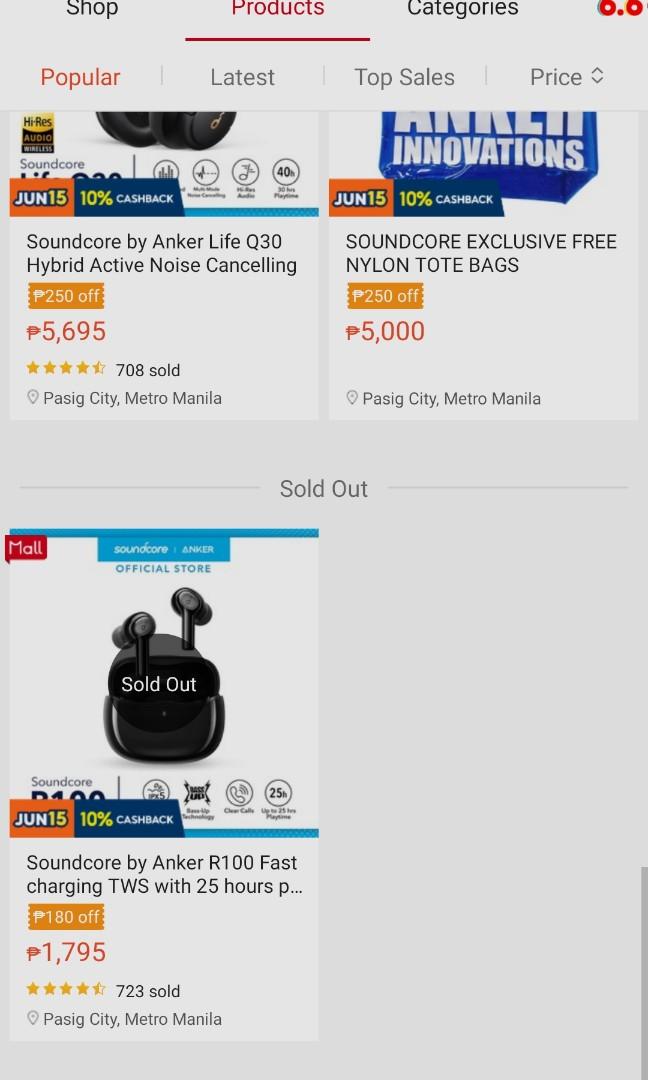The image appears to be a screenshot of a shopping app interface. At the top, a header labeled "Shop" is displayed, with the "Products" tab highlighted in red and underlined. To the right, there is another category labeled "Categories." In the top right corner, a small red icon resembling two eyes and a beak (perhaps an owl or bird face) is visible.

Below the header, a navigation bar displays four tabs "Popular" highlighted in a red-orange color, followed by "Latest," "Top Sales," and "Price" with up and down arrows indicating sorting options.

The main content showcases three products, with the images partially cut off. Starting from left to right:

1. **Product 1:**
   - **Name:** Soundcore by Anker Life Q30 Hybrid Active Noise Cancelling Headphones
   - **Discount:** ₱250 off
   - **Price:** ₱5,695
   - **Rating:** 4.5 out of 5 stars
   - **Sales:** 708 sold
   - **Location:** Kieg, Metro Manila (with a flag icon representing a specific location)

2. **Product 2:**
   - **Name:** Soundcore Exclusive Free Nylon Tote Bags
   - **Discount:** ₱250 off
   - **Price:** ₱5,000
   - **Rating:** (not provided)
   - **Location:** Pacific City, Metro Manila

3. **Product 3:**
   - **Name:** Soundcore by Anker R100 Fast-Charging TWS with 25 Hours Battery Life
   - **Discount:** ₱180 off
   - **Price:** ₱1,795
   - **Sales:** 723 sold
   - **Rating:** 4.5 out of 5 stars
   - **Location:** Pacific City, Metro Manila
   - **Status:** Sold Out

This detailed description covers the specific content and layout of the shopping app's interface, providing clear information on product details, discounts, and locations.